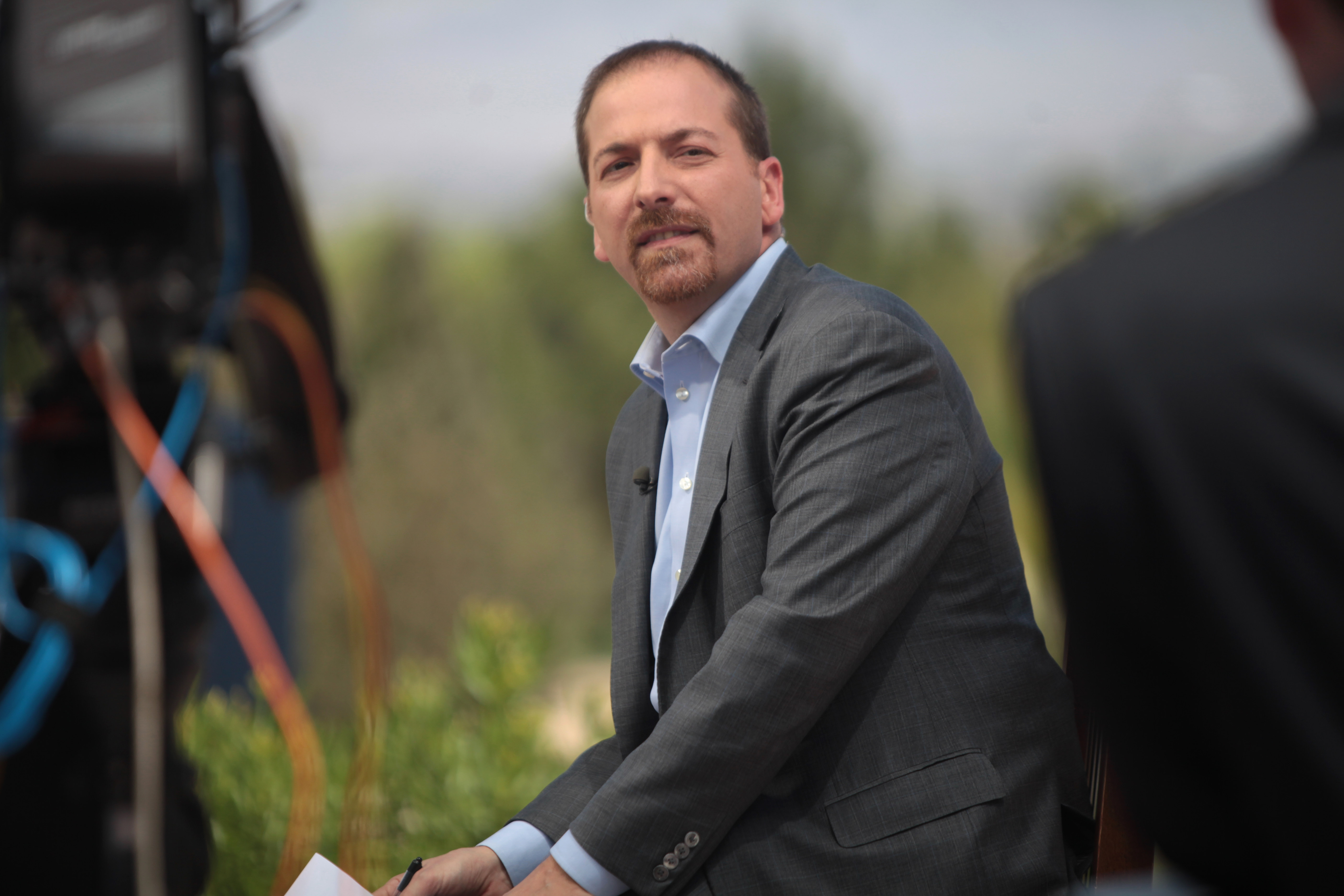This image features a man, identified as Chuck Todd from NBC News, likely known for his role on "Meet the Press." At the center of the frame, he is the sole element in sharp focus, while the background and other elements are blurred. Chuck has a very short, buzzy haircut with a receding hairline and a short brown goatee. He wears a gray suit jacket without a tie and a light blue button-down shirt. A small microphone is pinned to his jacket. His facial expression is quizzical, as he looks to the right with slightly beady eyes. His arms are positioned in front of him, possibly leaning, and he appears to be holding a piece of paper or pen, suggesting he might be looking at notes. The background features indistinct greenery, including trees and bushes, and there are blurred signs of filming equipment, like a camera and camera wires. Another person’s blurred shoulder is visible in the foreground, contributing to the impression that Chuck is engaged in a broadcast or an interview setting.